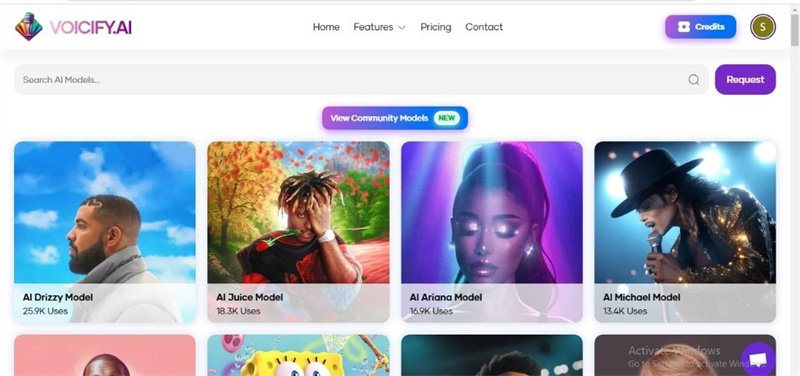The image showcases a landscape-oriented screenshot of a website related to artificial intelligence and voice technology, likely named "Voiceify.ai." The website features a top navigation bar set against a white background with a colorful, rainbow-like icon resembling a shell with a little head on top, followed by the site name "Voiceify.ai." The "V" in Voiceify is faint, with the text gradually darkening towards the "I."

Centered below the top bar are black navigation buttons labeled "Home," "Features," "Pricing," and "Contact." To the right of these buttons, there's a colorful oval, blending shades of purple and blue, with white text that reads "Credits." This oval also contains a circular icon, possibly an avatar, featuring a brown inner circle with a dollar sign or an "S" in the middle.

Beneath the navigation section, there's a gray search bar labeled "Search AI Models," accompanied by a purple "Request" button. Below this is a call-to-action bar with a purple and blue oval background that says "View Community Models" in white font.

The lower section of the page displays AI models styled after famous artists with their respective names and images. It lists "AI Drizzy Model" with an image of Drake, "AI Juice Model" featuring Juice WRLD, "AI Ariana Model" showcasing Ariana Grande, and "AI Michael Model" with an image of Michael Jackson. The images appear to be iconic photographs, possibly from their album covers or live performances.